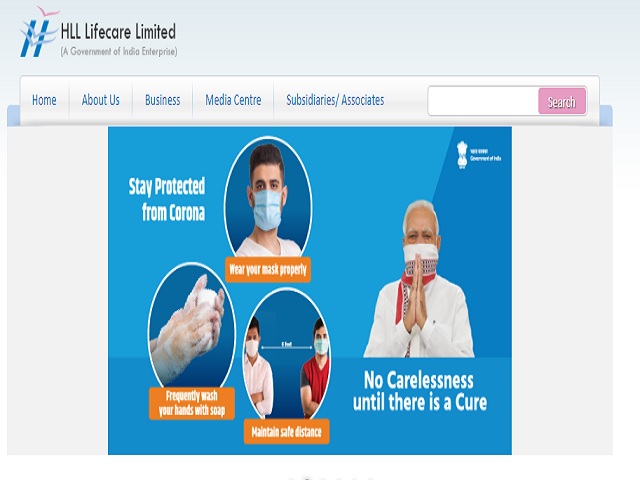The image contains several important elements arranged methodically to convey a message about COVID-19 safety measures. Towards the top of the image, there is a prominent blue box with the text "Stay Protected from Corona." Just below, in the center, is a circular image of a person wearing a surgical mask. 

Underneath this central image, there is an orange box with the instruction, "Wear your mask properly." To the left, another circle displays a person washing their hands, accompanied by an orange box that says, "Frequently wash your hands with soap."

Adjacent to this, there is a circle with two people standing side by side, both wearing face masks. The accompanying orange box instructs to "Maintain safe distance."

On the right side of the image, an elderly man with a bandana tied around his face is seen with his hands clasped together in a praying motion. An adjacent orange box cautions, "No carelessness until there is a cure."

Above all these elements, the text "HAL Life Care Limited, Government of India Enterprise" is prominently displayed. At the very bottom of the image, there is a navigation menu bar with options such as Home, About Us, Business, Media Center, Subsidiaries, and Associates.